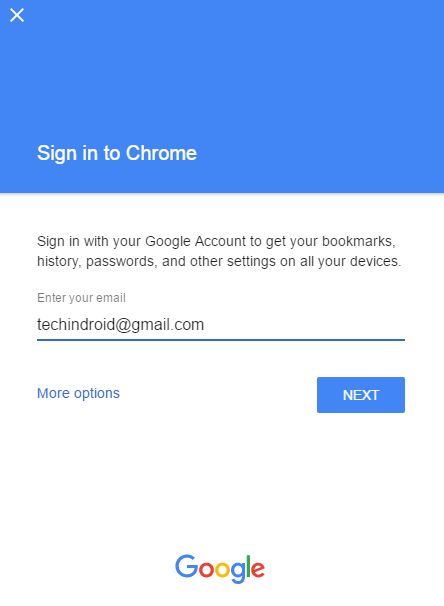The image captured from a phone screen displays the "Sign in to Chrome" page. The upper portion of the picture features a blue rectangle occupying the top space, within which a white 'X' is situated in the left-hand corner. Below this blue segment, the background shifts to white, prominently displaying the message "Sign in to Chrome" in white text. Underneath this header, additional text in black reads, "Sign in with your Google account to get your bookmarks, history, passwords, and other settings all on your devices," providing a brief explanation of the benefits of signing in.

Further down, in a smaller gray font, the text prompts users to "Enter your email." Below this prompt, the email address "techindroid@gmail.com" has been entered into the field. Underneath the email input field, a blue link labeled "More options" appears on the left side of the screen. To the right, the "Next" button is prominently displayed within a blue box, with the word "NEXT" in all-white, capitalized letters.

At the bottom of the screen, the multicolored Google logo is clearly visible, providing a familiar and reassuring element of branding.